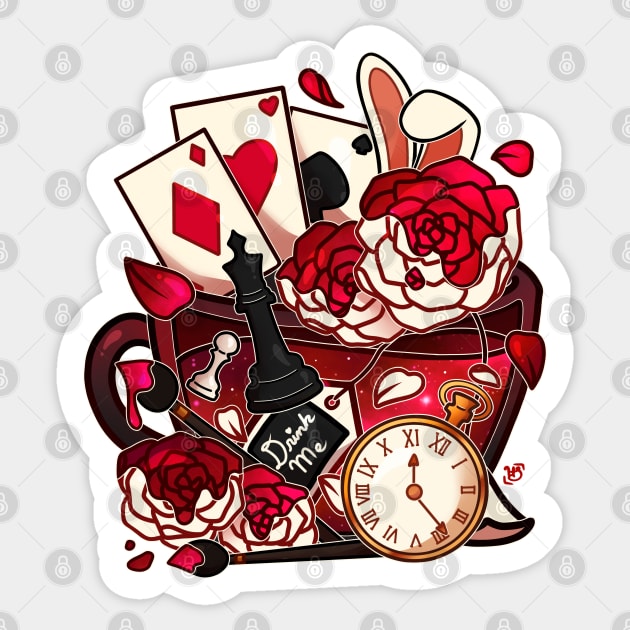This image is a detailed, computer-generated close-up of a sticker featuring a collection of whimsical illustrations inspired by Alice in Wonderland. Set against a white background with a subtle patterned watermark of small gray diamonds and disks, the sticker showcases a vibrant scene dominated by a red teacup. Peeking out from the teacup, which bears a tag reading "drink me" in elegant white cursive, are computer-generated playing cards – a diamond, heart, and spade. Surrounding the teacup are other notable elements from the story: partially painted red and white roses, a pocket watch with Roman numerals, and a pair of bunny ears. Additional details include chess pieces in front of the teacup, a couple of paintbrushes with red paint, and scattered rose petals. The entire scene captures the whimsical and fantastical essence of Alice in Wonderland.